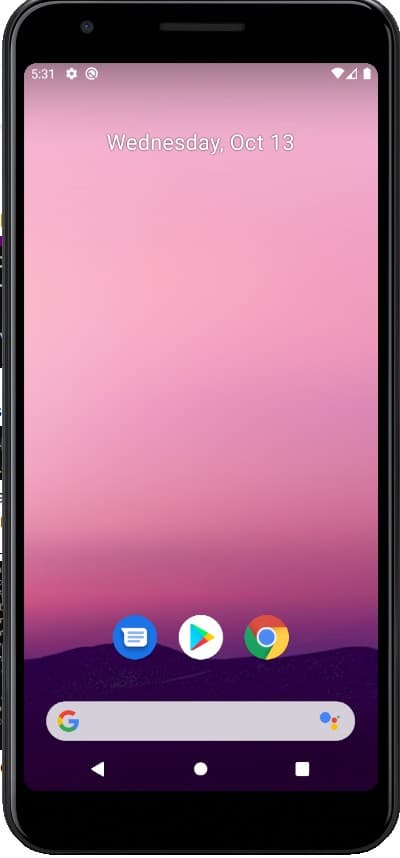The image shows a black smartphone displaying a screen with a predominantly pink background. At the top of the smartphone screen, the date "Wednesday, October" is written in white text. The lower portion of the screen features a slightly purple background.

Towards the bottom of the screen, there are three circular app icons arranged horizontally. On the left is the messaging icon, characterized by a blue circle with a white text message symbol. In the center is the Google Play Store icon, which consists of a white circle with a multi-colored triangle (green, blue, red, and yellow) pointing to the right. On the right side is the Chrome browser icon, depicted as a circle with interlocked segments in red, green, yellow, and white, and a blue circle in the center.

At the very bottom of the screen is the Google search box. The search box is white, featuring a multi-colored "G" logo (blue, green, yellow, and red) on its left side. To the right of the search box is the Google Assistant button, which is represented by four circles in green, red, yellow, and blue.